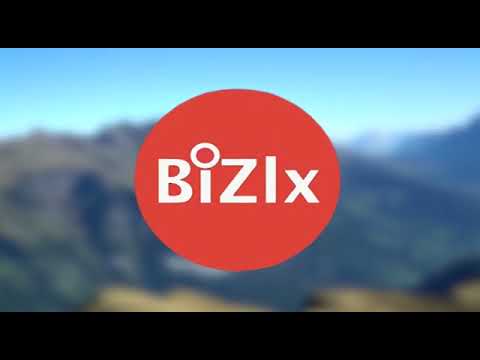This image, slightly wider than it is tall, features a central logo with letterboxed black borders occupying about 10-15% at the top and bottom. The focal point is a medium red circle centrally placed against a blurry background. Inside this red circle, white text reads "Bizlix" with a capital B, lowercase i with a larger circle dot, a capital Z, and lowercase l and x. The background, deliberately blurred to keep the focus on the logo, appears to depict a mountain range under a bright blue sky. The midpoint of the image transitions from dark brown to light brown, suggesting the ground beneath the mountain range.